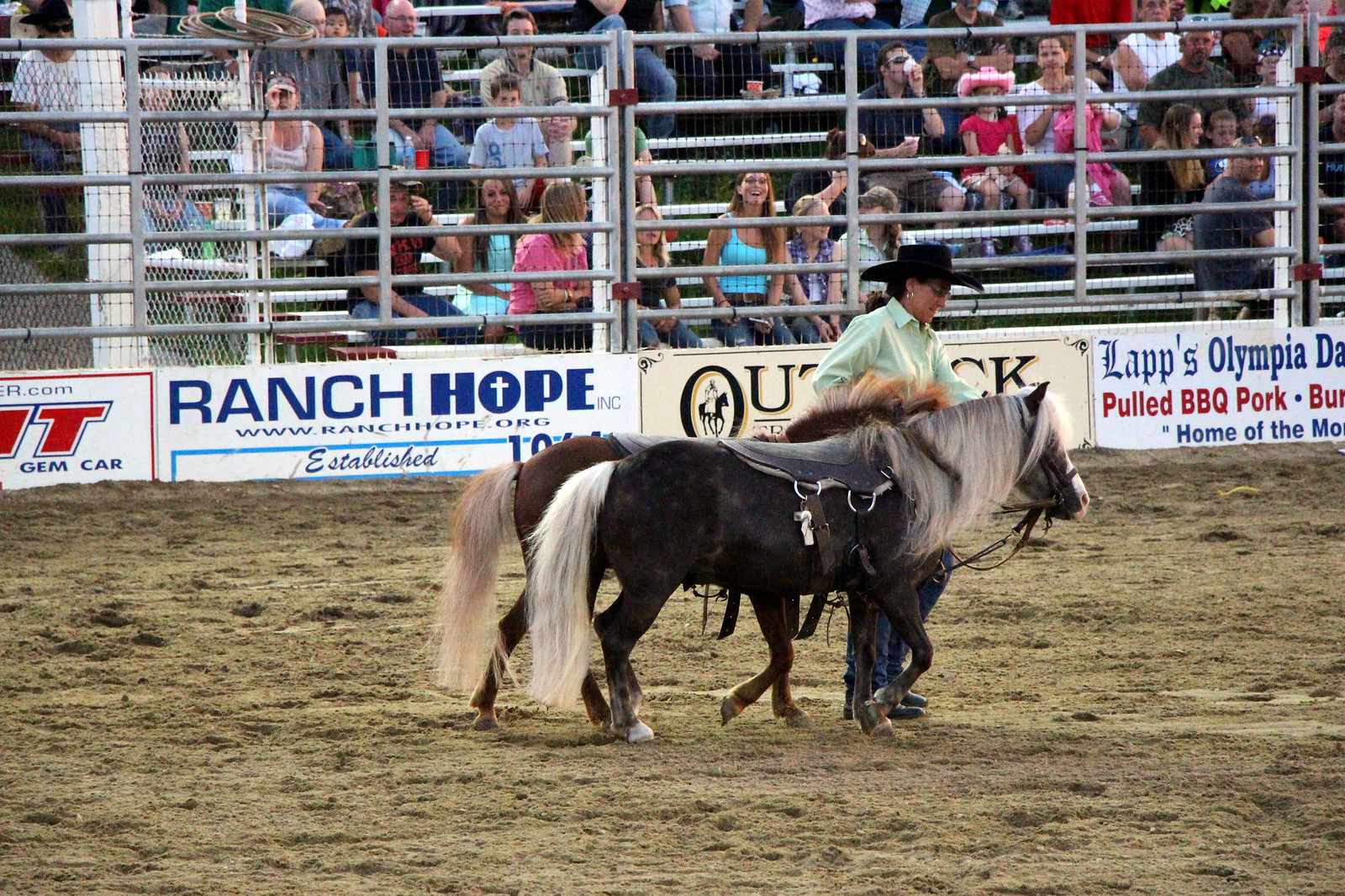This photograph captures a lively scene at a rodeo event. In the background, a crowd sits behind a tall fence adorned with various brand sponsor banners, including Ranch Hope, Last Olympia, Pool Park Pool, BBQ Pork, and the website www.ranchhope.org. In the foreground, a woman, dressed in a green shirt and black hat, guides two miniature horses—one brown and one black—across the muddy rodeo field. Both horses, distinguished by their very long manes and tails, are fitted with saddles. The engaging atmosphere of the rodeo is amplified by the lively audience visible in the stands.